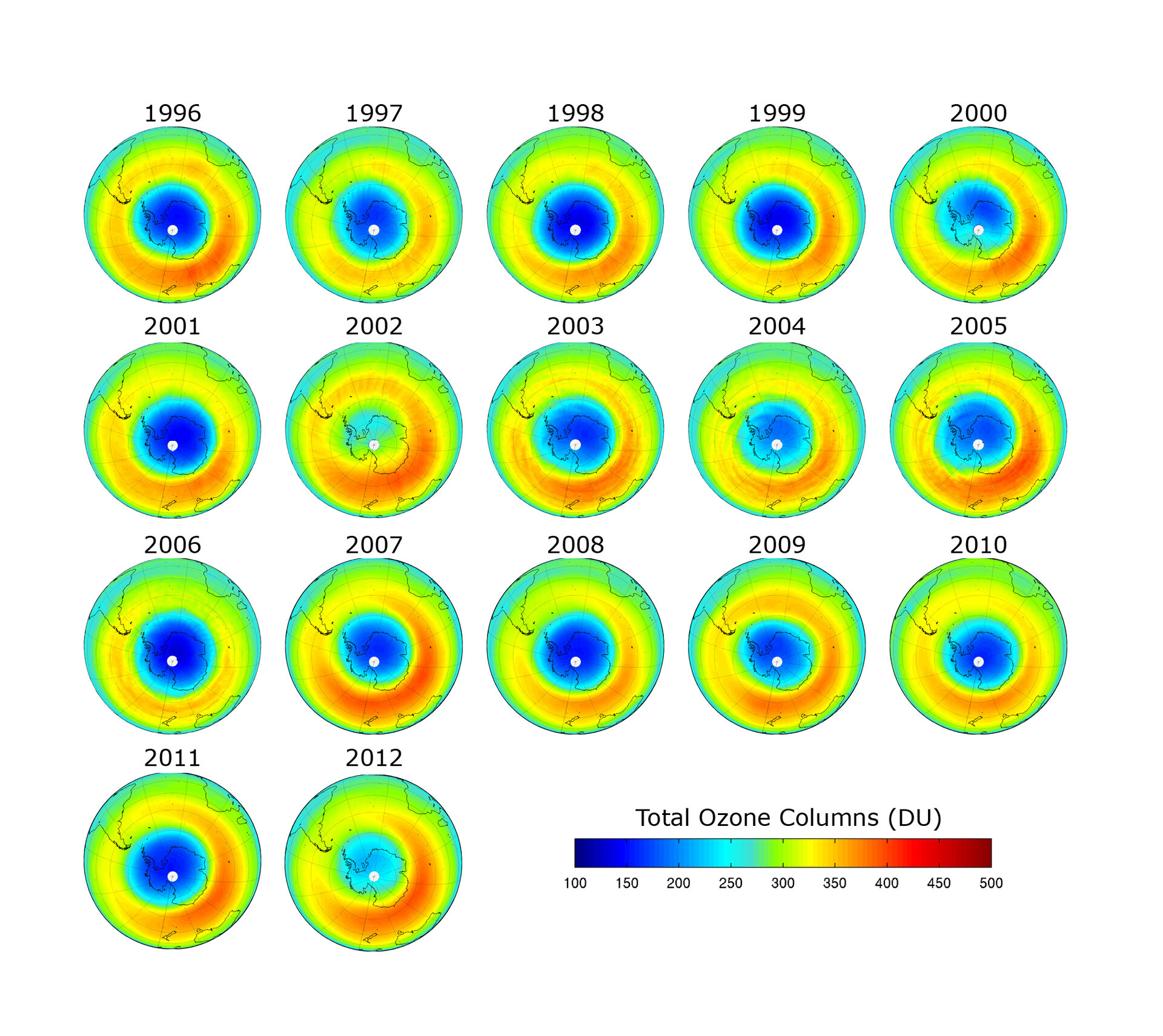This image features a white background displaying a series of 17 circles, arranged in three rows of five and one row of two. Each circle represents a specific year from 1996 to 2012, with corresponding labels placed above each circle. The topmost circle is labeled "1996," progressing through the years in sequence up to the last circle marked "2012."

Each circle exhibits multiple concentric layers, showcasing a color gradient that transitions from green at the outer edge to yellow, red, and then to various shades of blue, finally culminating in a white dot at the center. The colors within each circle illustrate the distribution and variation of ozone levels.

In the bottom right corner, there is a color-coded legend titled "Total Ozone Columns (DU)," which explains the color scheme used in the circles. The legend ranges from 100 DU (represented by dark blue) up to 500 DU (depicted in dark red). Intermediate values are marked by gradual shifts in color from dark blue to light blue, green, yellow, orange, and finally to dark red, correlating higher DU values with warmer colors.

This detailed visual chart allows viewers to compare the total ozone levels across different years, providing an intricate depiction of changes in the Earth's ozone layer from 1996 to 2012.